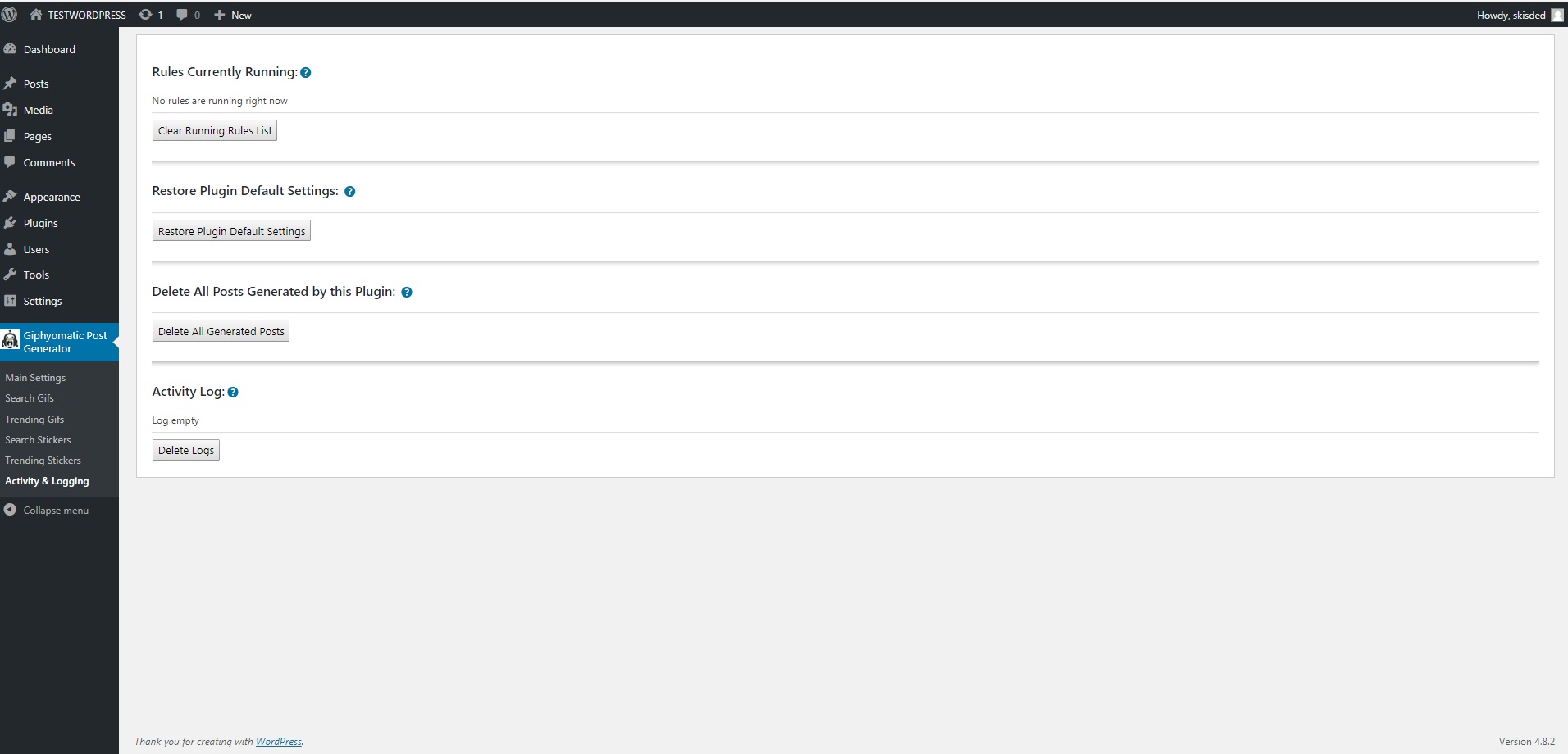The web page interface features a black bar at the top and a black sidebar on the left. The main window displays four options on a white background, each with a corresponding grey button featuring black text. The first option listed is "Rules - Currently Revising" followed by "Restore Plugins to Default Settings," "Delete All Posts Generated by This Plugin," and "Activity Log." On the black sidebar, one of the options is selected, highlighted with a blue rectangle. Text is small and challenging to read. In the bottom right corner of the page, the version number "4.8.2" is displayed.